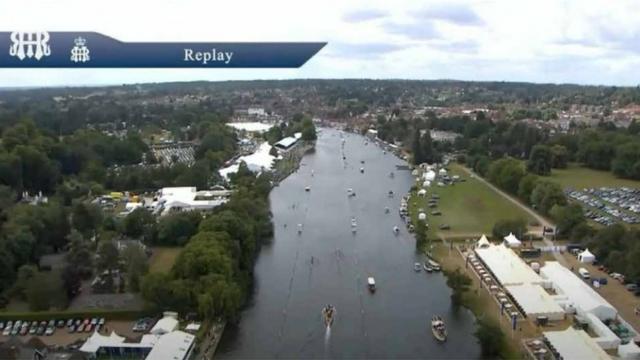The photograph captures a vibrant scene of a wide river or lake, bustling with boats, positioned centrally within the image. Framing the waterway are lush green forested areas and grass-covered expanses. On both sides, a small town or cityscape emerges, though only sparsely populated with buildings. 

The left side of the image features dense clusters of trees transitioning into distant structures as the river curves leftward out of sight. Meanwhile, the right side hosts a series of white buildings at the water’s edge, followed by parked cars on green lawns and a stretch of trees leading into an open grassy area. Further up, more buildings and trees dot the horizon.

Above this picturesque landscape, a white, cloud-laden sky suggests an overcast day. Dominating the top left corner, a bold sky-blue strip displays the word "REPLAY" in white font, accompanied by a few white symbols to its left. The overall color palette is rich and varied, with blues, greens, whites, and occasional splashes of yellow and red bringing the scene to life. The photograph evokes the atmosphere of a lively, perhaps competitive, marine setting, potentially capturing the essence of a motorboat race.